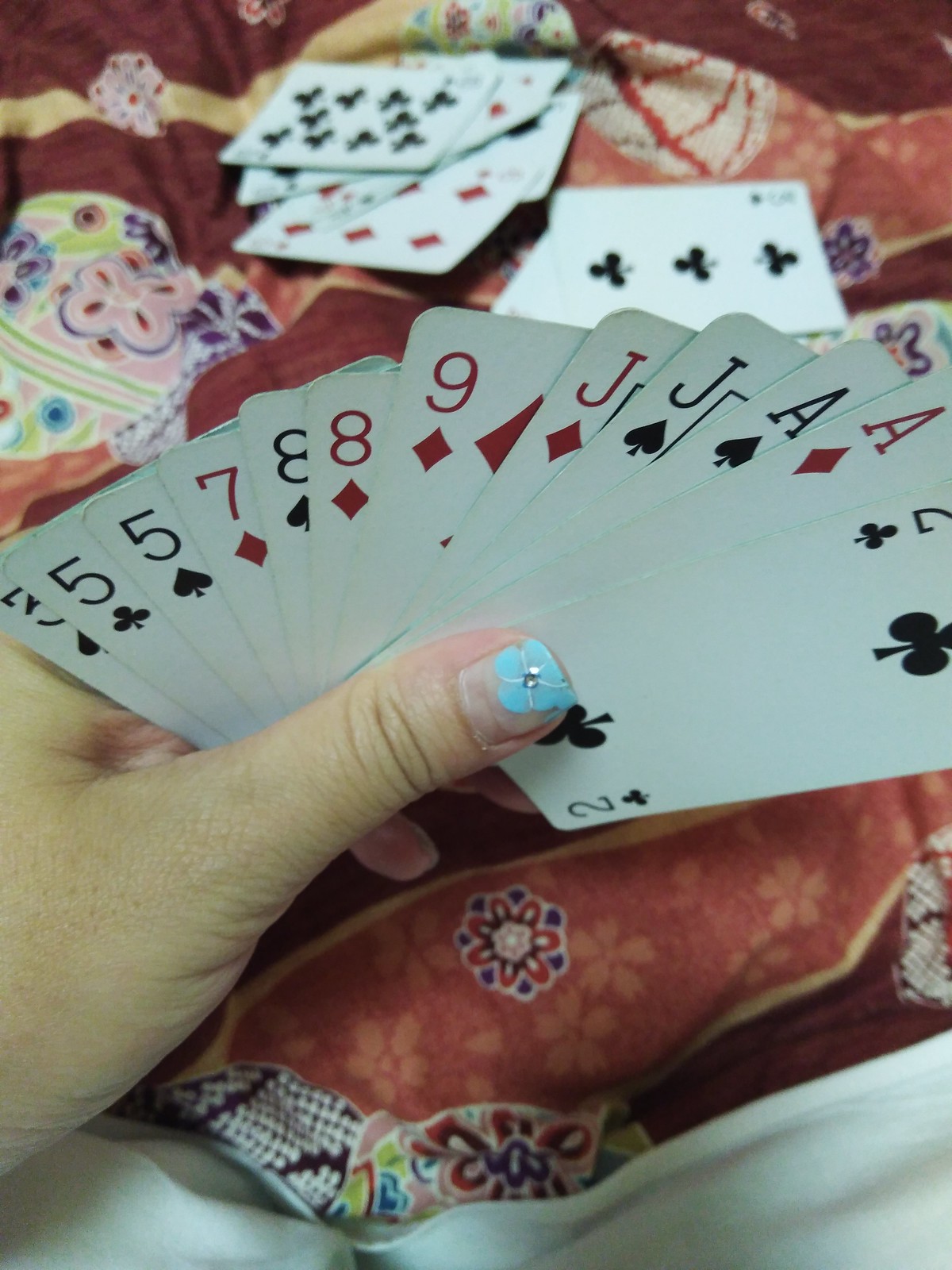In this vibrant and detailed image, a Caucasian woman is delicately holding a splayed deck of 12 cards in her left hand, skillfully displaying them in a semi-circular arrangement. Only her thumb, adorned with a beautifully painted blue flower nail art, is visible as it peeks from behind the fan of cards. The cards reveal only their top-left corners, adding an intriguing sense of mystery to the hand she holds. In the background, there is a rich, traditional cloth with intricate floral motifs in varied vivid colors, predominantly orange. The setting is further detailed with some face-up cards lying atop this floral fabric in the upper part of the image, indicating these are cards that have already been played. The stunning combination of the traditional cloth, the thoughtful manicure, and the compelling card arrangement creates a scene full of colorful details and cultural richness.